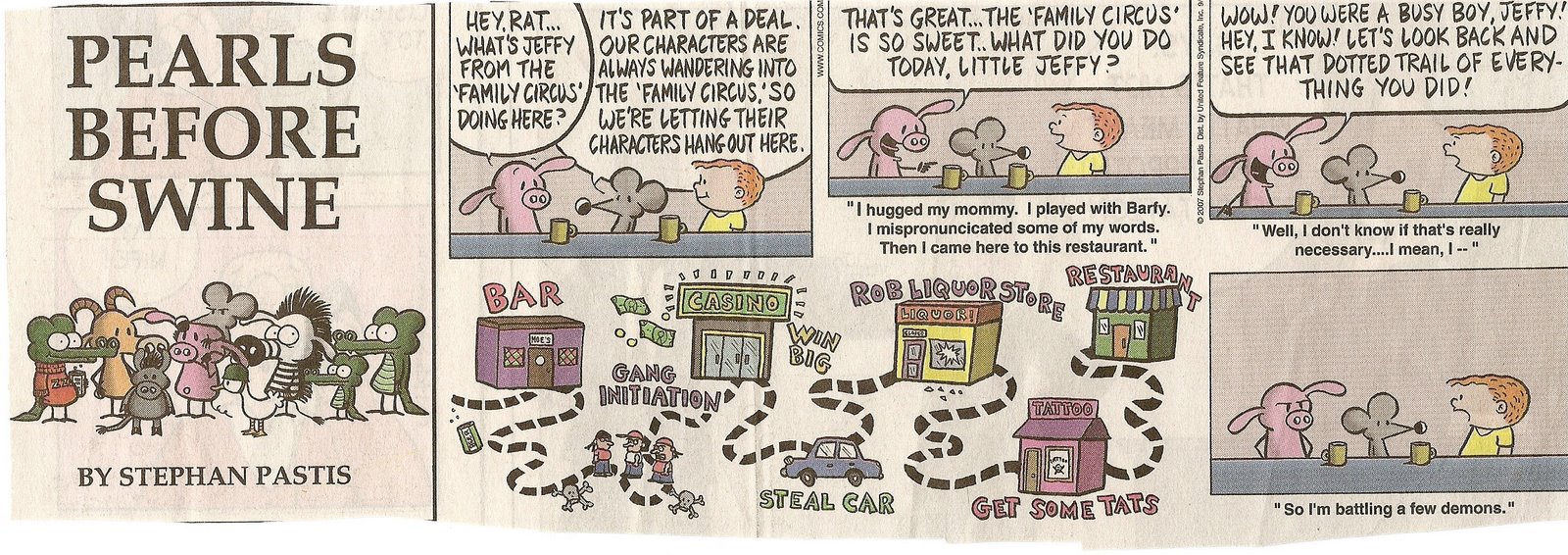This image is a vintage-style, full-color comic strip from the "Pearls Before Swine" series by Stephan Pastis, often seen in newspapers. The rectangular illustration is filled with a variety of animated characters including a crocodile, an elephant, a pig wearing a chef's hat, a bird, a hyena, and a zebra, all depicted in faded shades of pink, yellow, orange, black, white, green, and brown. At the very top left, the title "Pearls Before Swine by Stephan Pastis" is prominently displayed.

The comic strip features two main sections. The top section showcases a conversation between a pig, a mouse, and a boy named Jeffy from the "Family Circus" comic. The dialogue humorously depicts Jeffy recounting his day, saying he hugged his mommy, played with Buffy, and mispronounced words, illustrating the contrast between the wholesome 'Family Circus' world and the mischievous "Pearls Before Swine" universe.

The lower section of the strip depicts a sequence of events set in various locations represented by icons: a bar, a casino, a car, a liquor store, a tattoo shop, and a restaurant. The narrative follows the characters as they traverse from one location to another, ending with the pig, mouse, and boy again, with the caption, "So I'm battling a few demons," conveying the ironic undercurrent of the story.

Throughout, the comic cleverly juxtaposes the innocent world of Family Circus with the more cynical humor of Pearls Before Swine, creating a richly detailed and layered visual narrative.